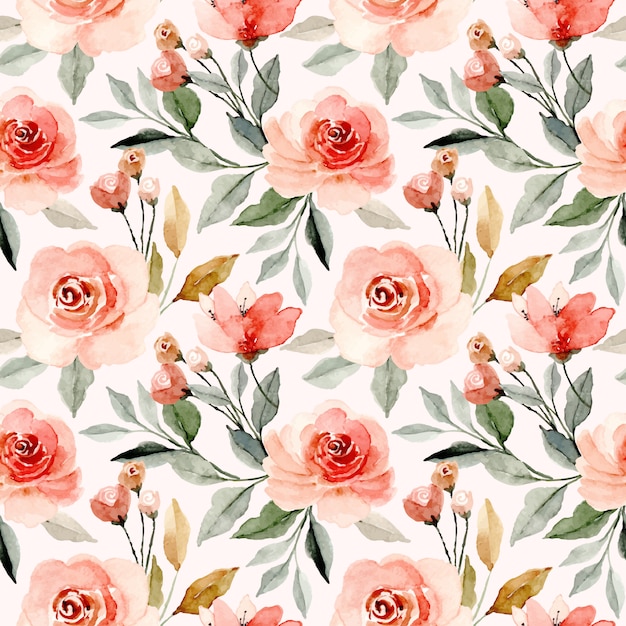The image depicts a digitally painted, symmetrical floral tapestry with a white backdrop. Prominently featured are large, open pink-peach roses arranged in alternating rows of four and three, with additional smaller, budding roses interspersed among them. The smaller roses appear in pink and a yellowish hue. Light green leaves accompany the flowers, some of them showing signs of browning or dying, adding a touch of realism to the arrangement. The design also includes some brown, blue, and green elements, possibly leaves or small undeveloped flowers, enhancing the overall texture and depth. This detailed and vibrant floral pattern could serve as a decorative background, tablecloth, or wallpaper.